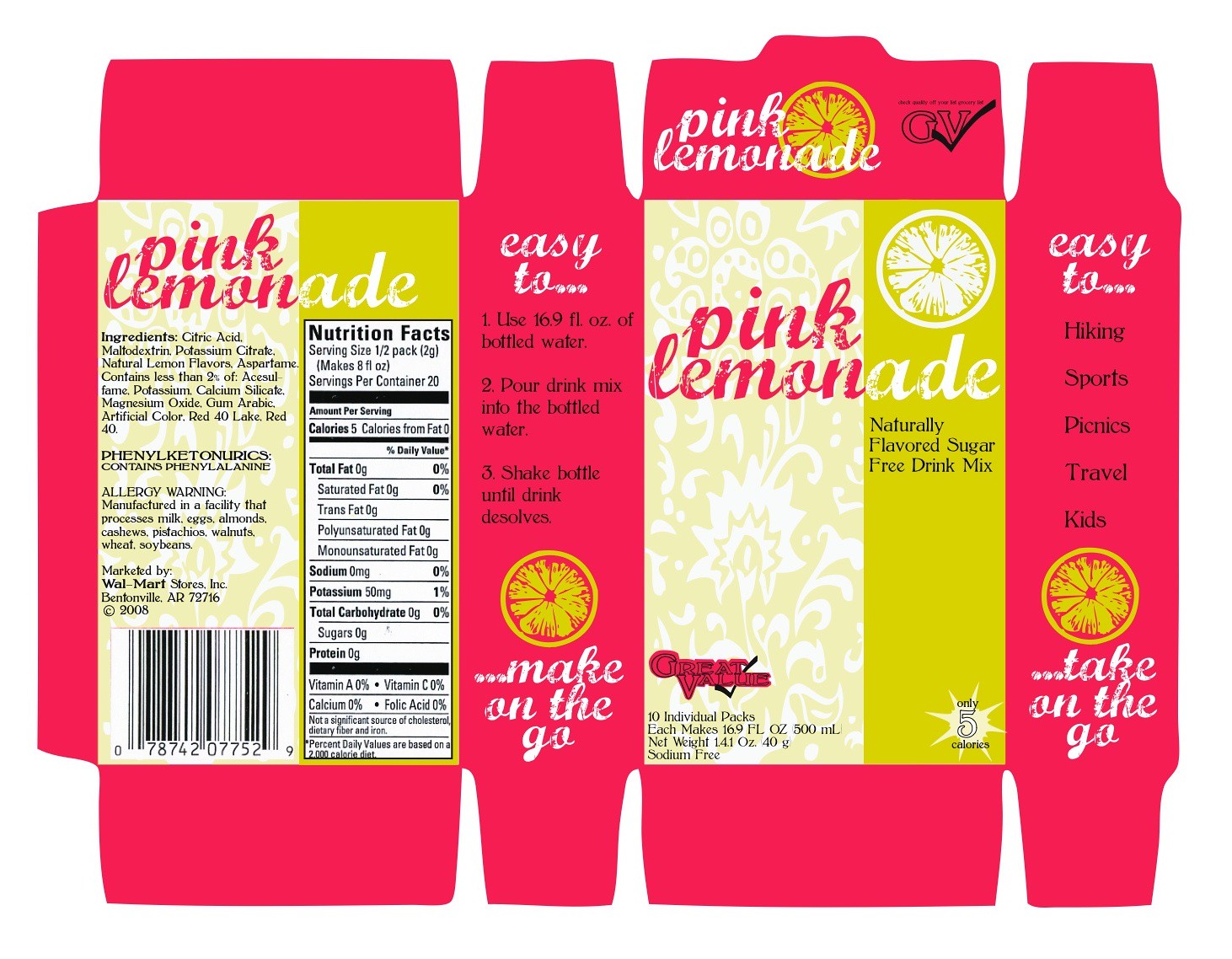The flattened drink mix box displays a variety of informative and promotional elements. One prominent side features the product name "Pink Lemonade" in black font against a backdrop of pink and white. Beneath this, there is a list of ingredients, followed by an allergy warning in black font, cautioning that the product was processed in a facility that handles milk, eggs, almonds, cashews, pistachios, walnuts, wheat, and soy. Additionally, the packaging indicates that this product is sold exclusively at Walmart stores. A black and white barcode is also visible on this side.

On another side of the box, a white label displays detailed nutrition facts in black font. Adjacent to this section, in white font, the box declares the product is "easy to make," accompanied by a graphic of a yellow lemon. 

Elsewhere on the packaging, pink and white fonts are used alongside more black text, announcing that the drink mix is naturally flavored and sugar-free. Gold lemon graphics add a splash of color, enhancing the overall aesthetic of the packaging. Various other informational texts are printed in both white and black fonts throughout the design.